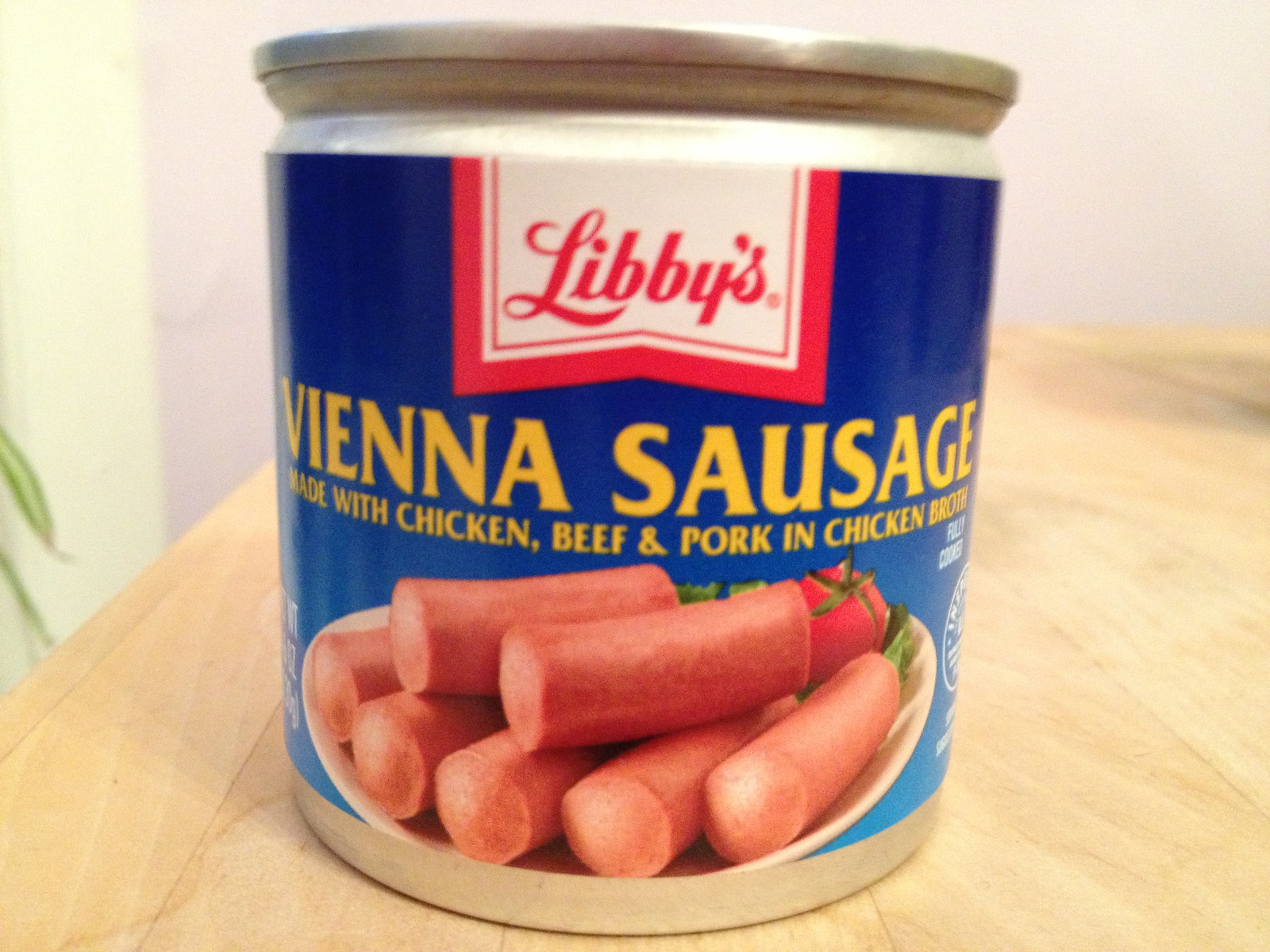The image prominently features a can of Libby's Vienna Sausage, situated centrally on a light wood grain table background. The cylindrical aluminum can, topped with a silver lid, showcases a striking blue label. A white tab with a red, indented border displays the brand name "Libby's" in red cursive font. Just below, large yellow letters announce "Vienna Sausage," followed by a smaller yellow text detailing that it's "Made with Chicken, Beef, and Pork in Chicken Broth." A detailed image on the can's label highlights a plate of pinkish, cylindrical Vienna sausages, resembling short hot dogs, accompanied by a ripe red tomato and a small sprig of green vegetation. The overall scene is complemented by an off-white or light lavender wall in the background, with a hint of white wooden surface and two green leaves from a variegated plant appearing to the left of the can. Partially visible on the right, there's also a USDA or food service label.